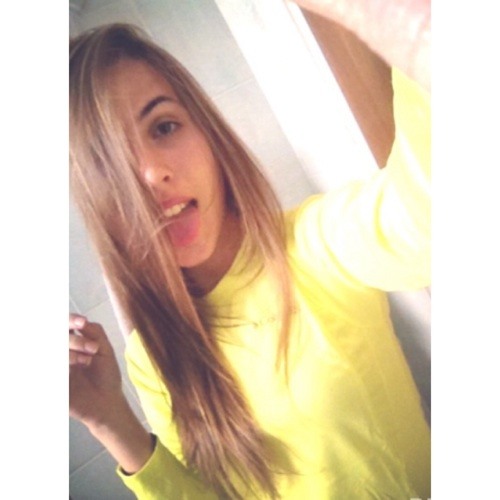The image features a young woman, likely in her late teens or early 20s, with long, straight, brownish-blonde hair that extends past her bosom. Her skin tone is light and she has dark brown eyebrows. She is facing the camera, possibly taking a selfie, indicated by her extended left arm holding the phone, which is out of frame. Her right arm is bent with fingers curled, and she appears to be enjoying herself as she has a playful expression with her mouth open, displaying her top row of teeth and her tongue which sticks out. She is wearing pink lipstick and a long-sleeved yellow shirt. The background is grayish white, suggesting a bathroom setting with tiled walls, and in the upper right corner of the image, there are hints of a door frame or another structure with brown and white coloring. The majority of the image is filled by her face and upper torso.